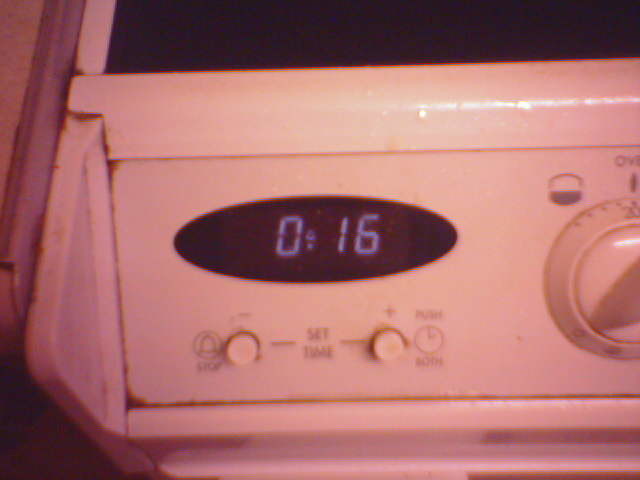The image depicts the front panel of a poorly maintained stove or oven with a focus on a timer and control dials. On the right side, there is a greasy and dirty dial labeled "OVE," presumably short for "oven," which is currently set to 200-something degrees. To the left of this dial is a black elliptical digital display showing "016" in bright blue digits. Below the display are two circular buttons – the left one marked with a bell icon and labeled "stop," and the right one labeled with a clock icon and "push." Between these buttons, the words "set time" are printed. At the top middle, part of a black stovetop is visible, and a grayish countertop borders the upper left corner. The stove's overall condition emphasizes its urgent need for cleaning.